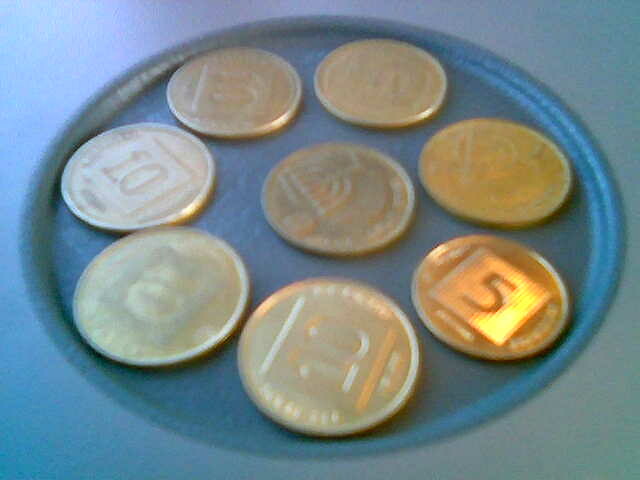This photograph features a teal plate with a flat bottom and a two-tiered rim, placed at the center of a background shaded with a gradient of blue, gray, and purplish hues, creating a sense of depth and dimension. Upon the plate, there are eight coins: seven positioned in a circle along the outer edge and one placed in the center. The coins appear to be of foreign origin, with several displaying the number ten and one prominently showing the number five. The coins are mostly brass with one notably shinier and silver in appearance. The image is slightly out of focus, making the finer details of some coins difficult to discern.